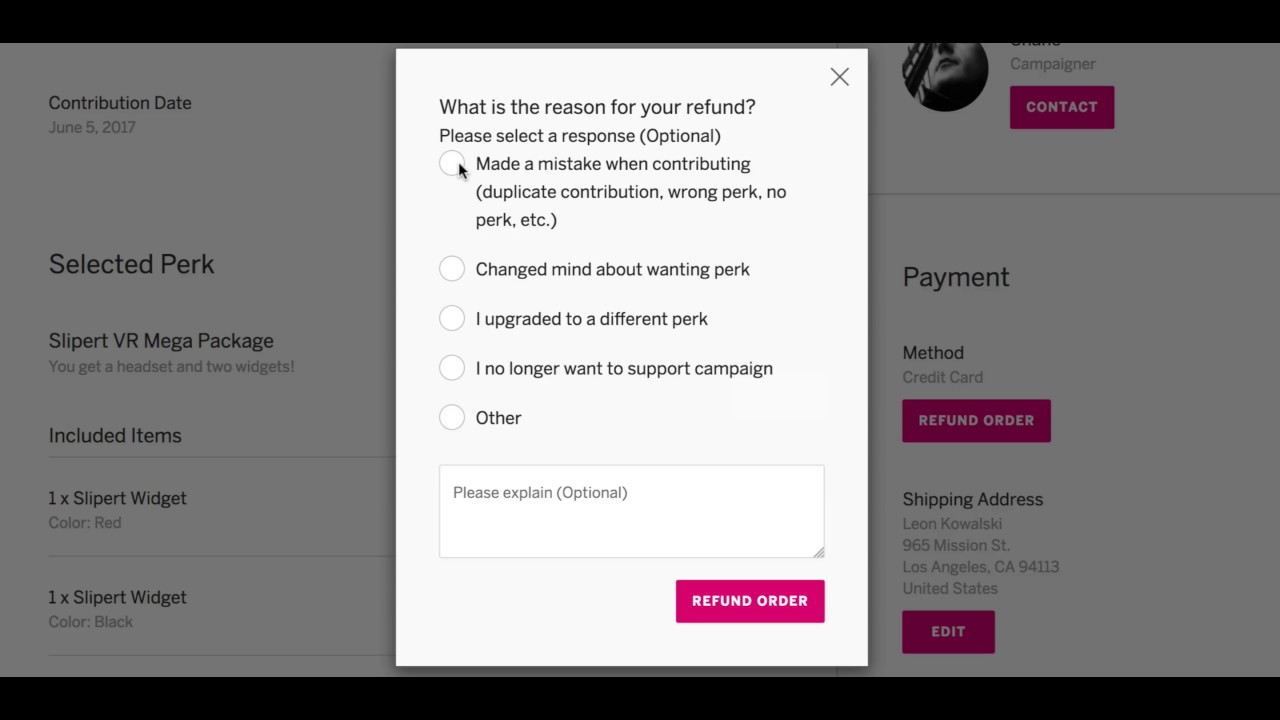A detailed screenshot depicts a VR-related webpage where a user is in the process of requesting a refund. The website features thin black bars at the top and bottom. 

In the upper left corner, "Contribution Date: June 5th, 2017" is displayed. Below, it mentions "Select Perk: Slipperd VR Mega Package," which includes a VR headset and two widgets. The section further lists the included items: one red Slipperd widget and one black Slipperd widget.

In the upper right corner, there is a profile picture adjacent to the name "Campaigner" with a "Contact" button and the payment method noted as "Credit Card." A prominent "Refund Order" button is situated just below.

Further down, the shipping address is provided as: Leon Kowalski, 965 Mission Street, Los Angeles, California, 94113, United States, with an "Edit" button to the right, albeit half-grayed out.

Centrally, a pop-up prompts the user with "What's the reason for your refund? Please select a response (optional)." The mouse cursor is hovering over the first option, "Made a mistake when contributing." Other selectable reasons include "Duplicate contribution," "Wrong perk," "No perk," "Changed mind about wanting perk," "I wanted a different perk," "I upgraded to a different perk," "I no longer want to support the campaign," and "Other." There is also an optional "Please explain" field. The pop-up concludes with a prominent pink "Refund Order" button.